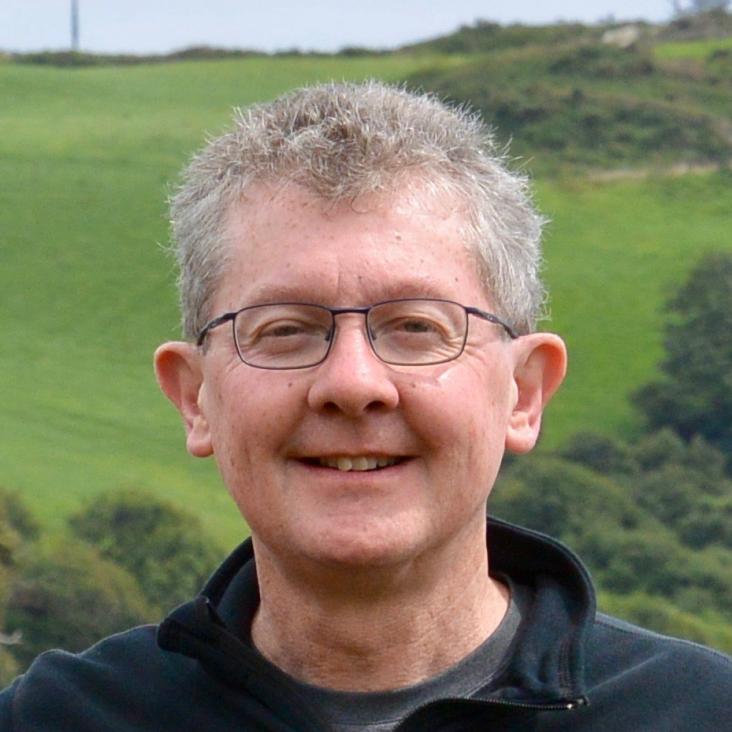The image is a detailed outdoor portrait of an elderly white man, likely in his late 50s or 60s, captured on a cloudy day. He has short, grayish-brown hair that leans more towards gray, marked with signs of aging such as crow’s feet and prominent wrinkles at the edges of his eyes when he smiles. His face features dark brown spots or freckles, and he wears black-rimmed spectacles. His ears fold outward towards the top. He has a cheerful expression, revealing slightly yellowed and crooked teeth. The man is dressed in a dark-colored, possibly blue, unzipped sweater, under which you can see a bit of a gray shirt. The background showcases a smooth, rolling grassy hill with patches of green bushes and small trees, adding a serene, natural backdrop to the portrait.